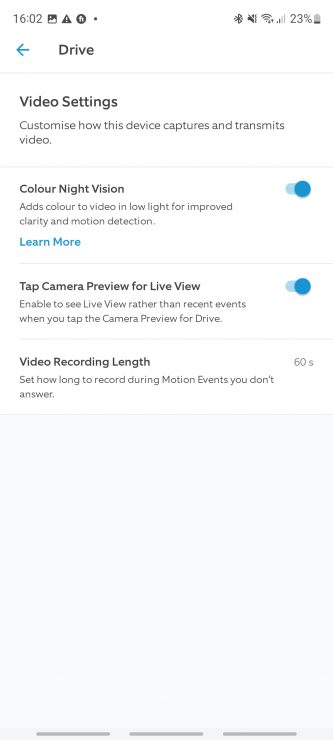The image is a detailed smartphone screenshot with a white background. At the top left corner, the time reads "16:02", while on the right side, the signal strength shows two out of four bars and the battery indicator displays 23% remaining. Below this, a blue arrow pointing left accompanies the word "Drive" in bold black letters.

The main section of the screenshot is divided by thin, light gray lines into several segments. At the very top, the words "Video Settings" are written in black. Directly below, in smaller gray text, it says "Customize how this device captures and transmits video."

The next section is titled "Color Night Vision" in black text, with a description underneath in gray: "Add color to video in low light for improved clarity and motion detection." Beside this description, a blue toggle switch indicates that the feature is turned on. Below these details, the phrase "Learn more" is written in blue text.

The final section is labeled "Tap Camera Preview for Live View" in black text, with a corresponding blue toggle switch on the right side, also turned on.